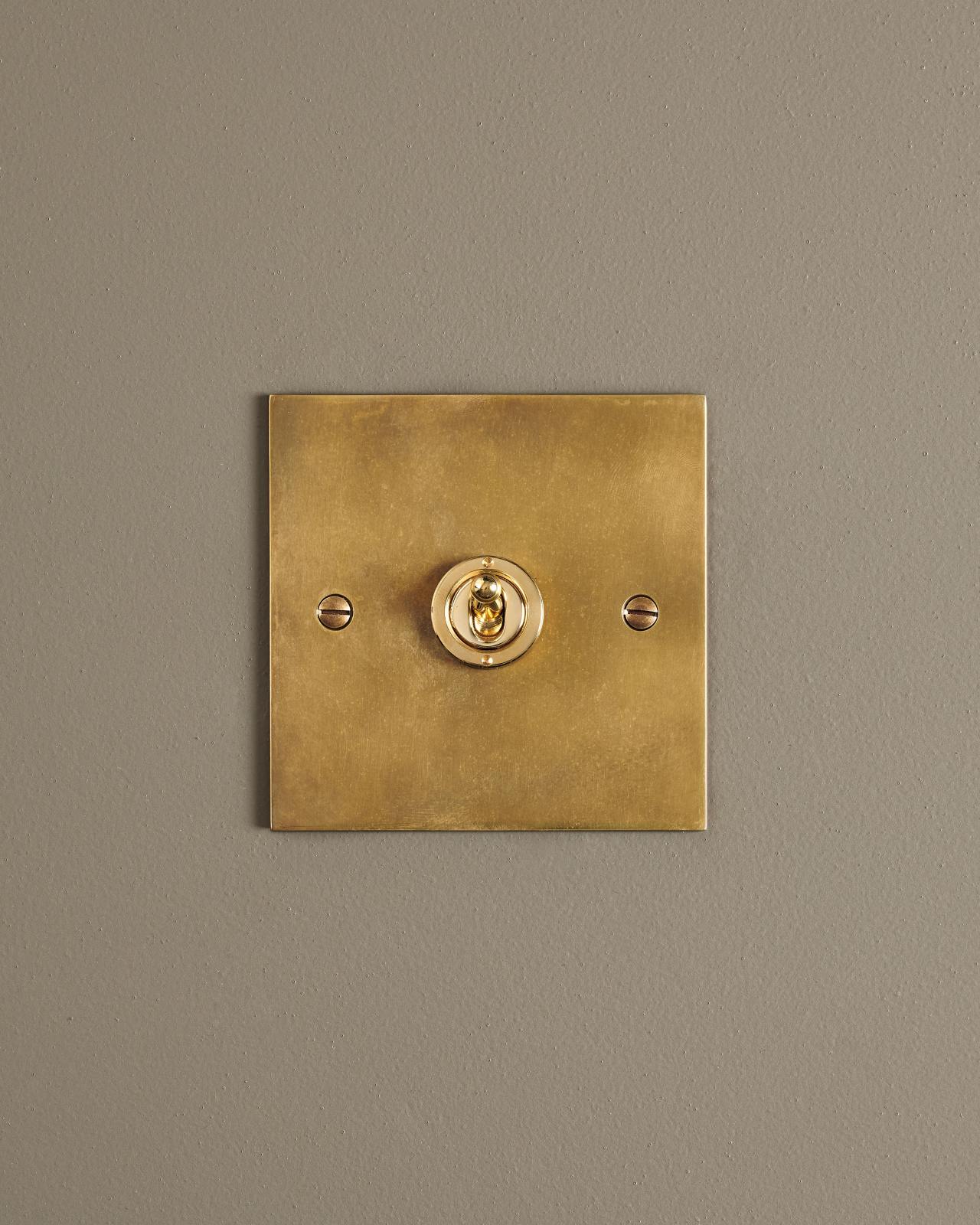This image depicts a gold metal plate mounted on a gray wall. The plate features two screws, positioned horizontally on the left and right sides. Both screws are either white or gold, shiny, and have their flat-head slots aligned horizontally. In the center of the plate, there is a round, shiny gold circle with a protruding gold knob, likely associated with a light switch. The surface of the plate has an ombre effect, showcasing varying shades of pale gold and darker grayish hues, adding a delicate texture to its finish. There is no text visible in the image.